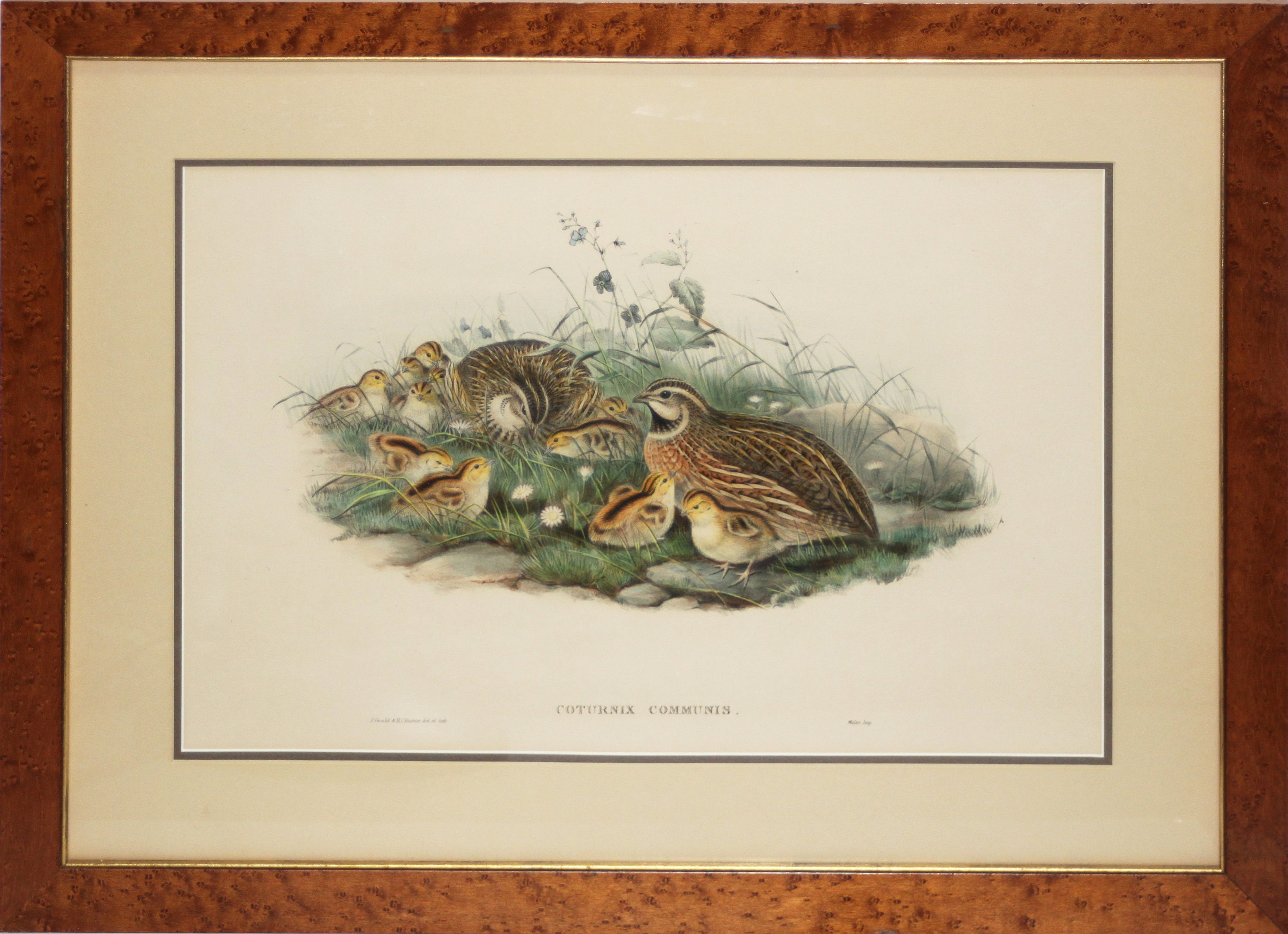This photograph captures a framed watercolor painting of two adult quail, Coturnix communis, surrounded by their group of chicks, which range from 10 to 11 in number. The quail family is depicted nestled in a meadow environment with muted, pastel colors: the vegetation appears in shades of light green, and the quail are illustrated in hues of gold, brown, black, and red. The foreground is populated with small rocks and three yellow and white flowers, while taller blades of grass in the background seem to sway, adding a sense of movement. One adult quail looks upwards, showing the side of its face, while the other peers down into the grass. The painting fades seamlessly to a white background at the edges. The artwork is matted in gray and taupe, and framed in a reddish-golden-brown textured wood. Beneath the painting, the text "Coturnix communis" is inscribed, likely identifying the species.